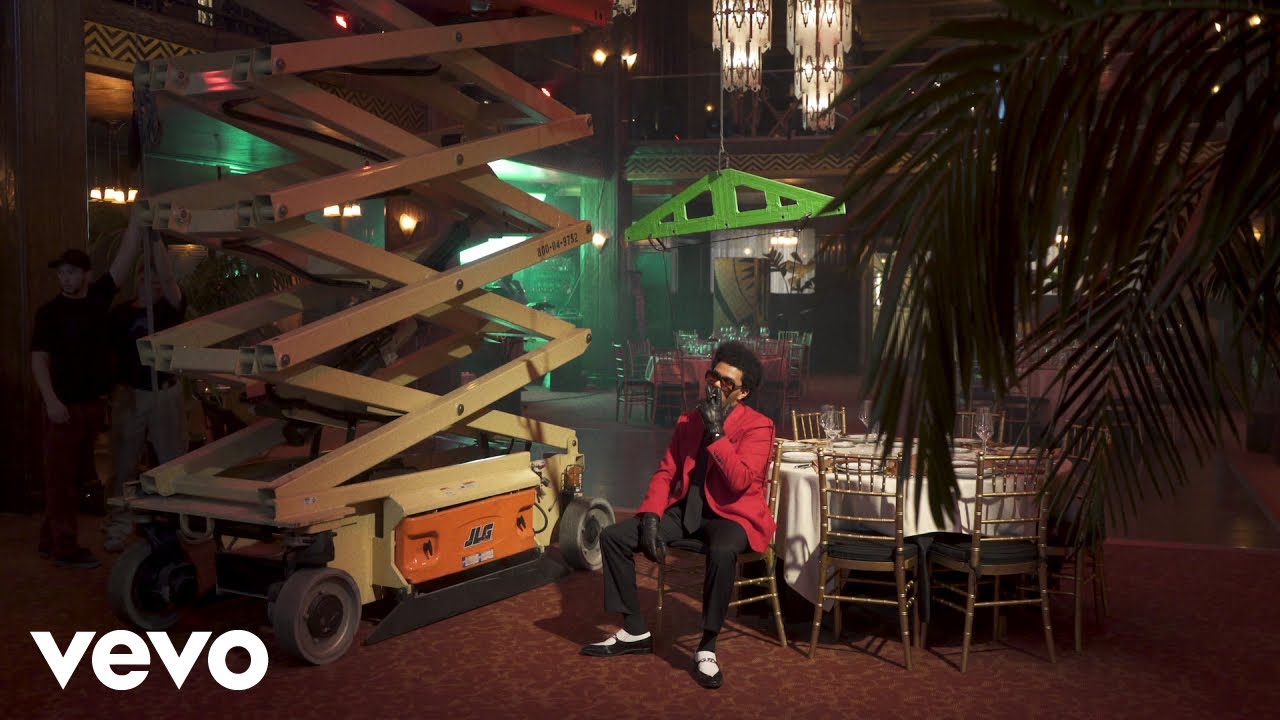This vivid color photograph captures the interior of a two-story coffee shop or restaurant, characterized by a sense of elegance and complexity. Dominating the center is an African-American man, clad in a striking ensemble of a red jacket, black pants, a black tie, white and black two-toned shoes, and black gloves. He's wearing sunglasses and smoking a cigarette, exuding a cool and relaxed demeanor as he sits on a wooden chair designed to resemble a cane.

To his right, a round table draped in white tablecloths is set with plates and surrounded by chairs, suggesting a dining setup ready for guests. To his left, a bright yellow scissor jack with an orange and yellow base extends beyond the photograph’s upper frame. The text "JLG" is visible on the side of the scissor jack, hinting at its industrial purpose, possibly for adjusting the numerous lights or hanging decorations. Two men, dressed in black tops and light-colored pants, appear to be operating this equipment.

Above the man and toward the photograph's center, a green triangular metal piece is suspended from the ceiling, adding to the intricate decor. The background reveals more tables set for dining, a visible balcony, and a grand chandelier hanging above the man’s head. Additional lights and hanging palms accentuate the upper right corner of the image, adding lush greenery to the setting. The floor features a red pattern, contributing to the venue's aesthetic. Prominently, the word "VIVO" is displayed in large white text at the lower-left corner, slightly below the man, adding a branding element to the scene.